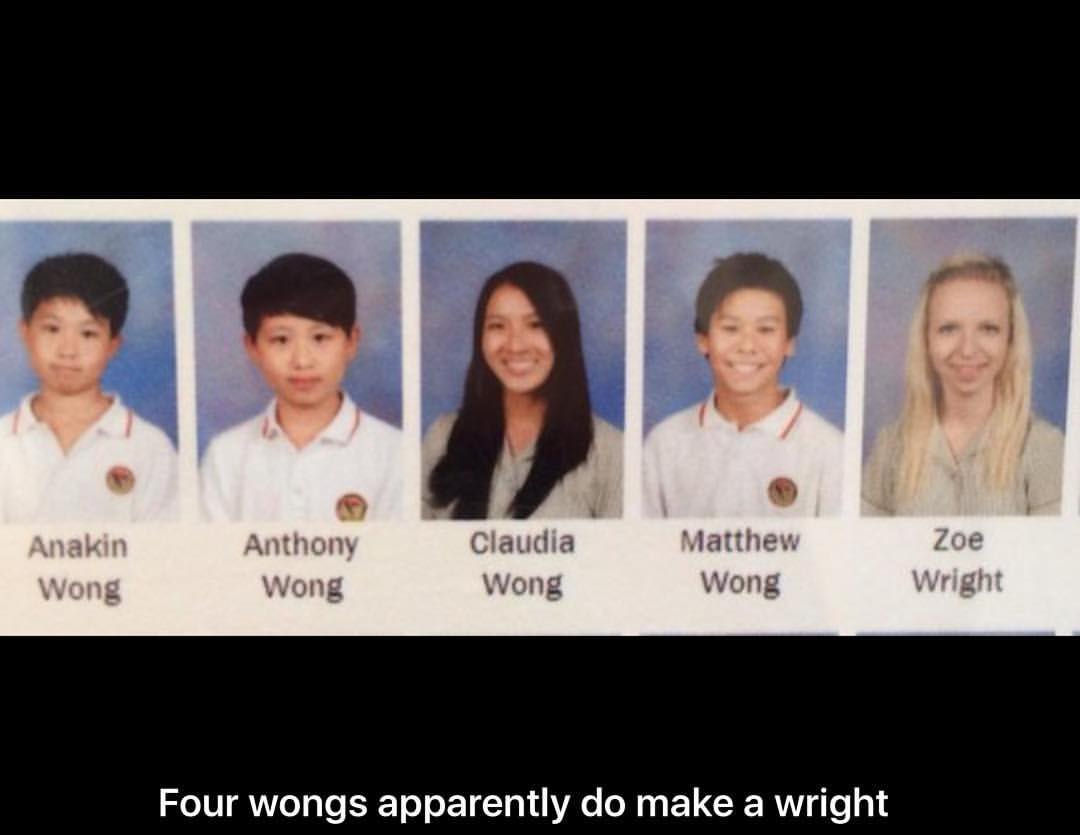The image appears to be a partial page from a school yearbook with a humorous, albeit controversial, meme-like caption. The backdrop is entirely black, and five student photographs are aligned in a row from left to right. The first four students share the last name Wong and are identified as Anakin Wong, Anthony Wong, Cataleya Wong, and Claudia Wong, all appearing to be of Asian descent. The fifth student, Zoe Wright, stands out with her blonde hair and Caucasian background. Beneath the row of photographs, white text on a black frame reads, "Four Wongs apparently do make a Wright." The joke references the pun in their last names but may come off as insensitive and not very clever, especially considering these students appear to be around seventh grade.